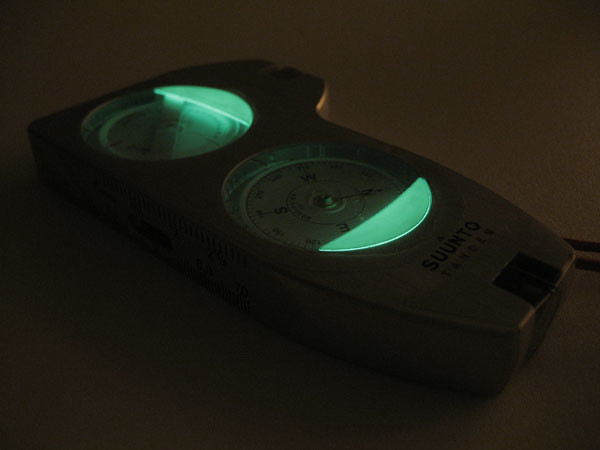A dimly lit photograph captures a digital object resembling a gauge, positioned diagonally with its bottom at the lower right corner and top at the upper left. The background gradient shifts from an extremely dark brown in the bottom left corner to a slightly lighter tint towards the top, yet remains predominantly dark and shadowy, cloaking much of the image in obscurity.

In the top right quadrant, extending into the central upper portion, a protrusion disrupts the otherwise rectangular form of the device. Adjacent to this protrusion, a glass-covered dial with an eerie greenish hue emanates light from its right side. Though there's writing or numbers on the dial's darkened face, they are unreadable due to the shadows.

Below this dial, another glass-covered window illuminates the very bottom edge with a striking lime-green light, revealing a set of numbers and a gauge resembling a clock face, though it's evidently not a timepiece. The dark housing of the object bears a title just above the bottom right corner, the text "S-E-U-N-T-O" (likely "Suunto"), offering a vague hint to its identity while leaving its function ambiguous.